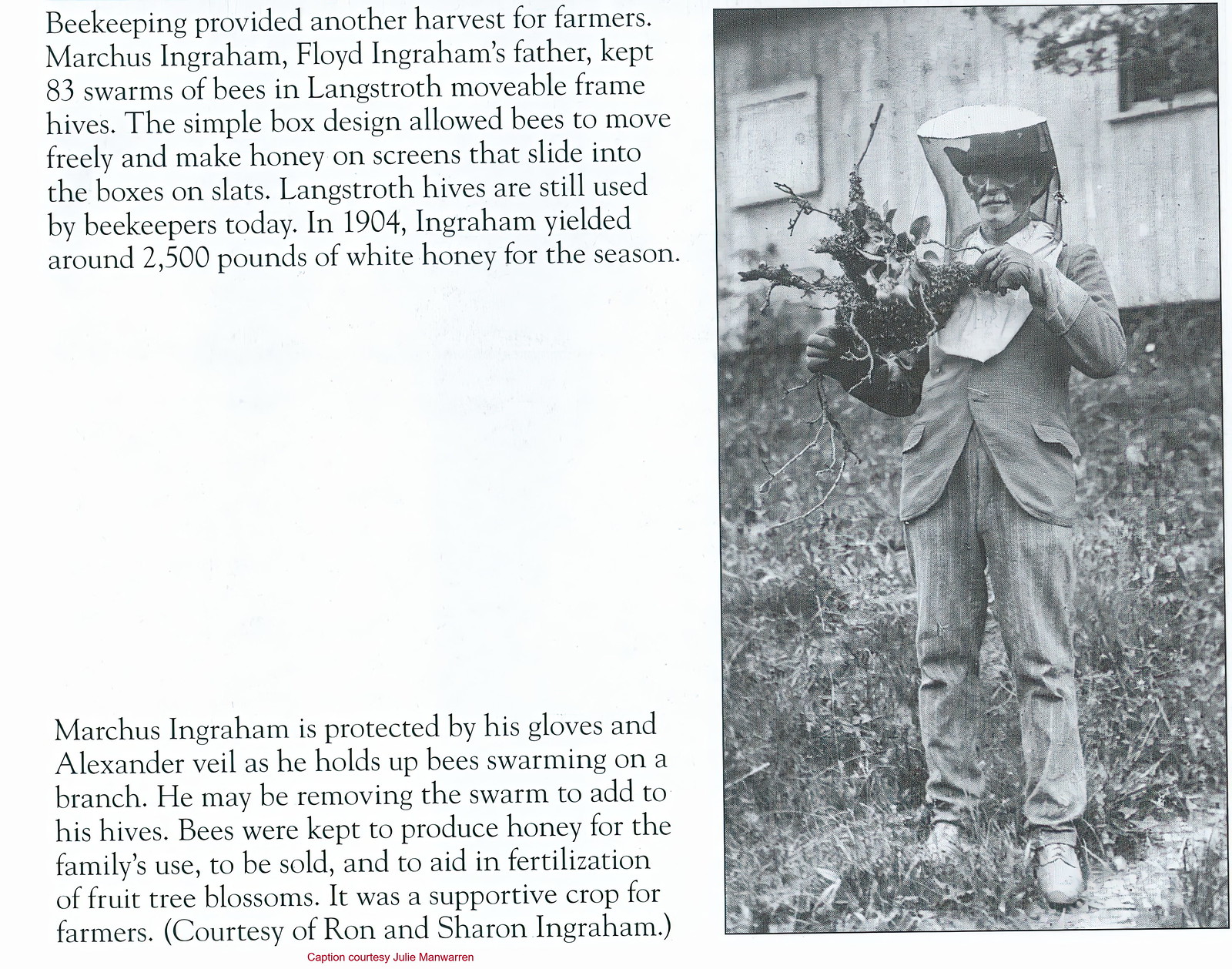The black-and-white photograph captures an early beekeeper, Marcus Ingraham, dressed in traditional protective attire, including an Alexander veil and gloves. He stands on a grassy slope holding a branch with a bee swarm, possibly being removed to add to his hives. Marcus, the father of Floyd Ingraham, managed 83 swarms in Langstroth movable frame hives, which allowed bees to move freely and produce honey on screens that slide into the boxes on slats. This design is still in use today. In 1904, Marcus Ingraham's hives produced approximately 2,500 pounds of white honey. Behind him, a building forms the backdrop of the image, contributing to the historical context. The textual narrative on the left emphasizes the significance of beekeeping as a supplementary harvest for farmers, aiding in honey production, family use, sale, and the fertilization of fruit blossoms. The image and text combine to depict beekeeping's importance in early 20th-century agriculture. Courtesy of Ron and Sharon Ingraham.